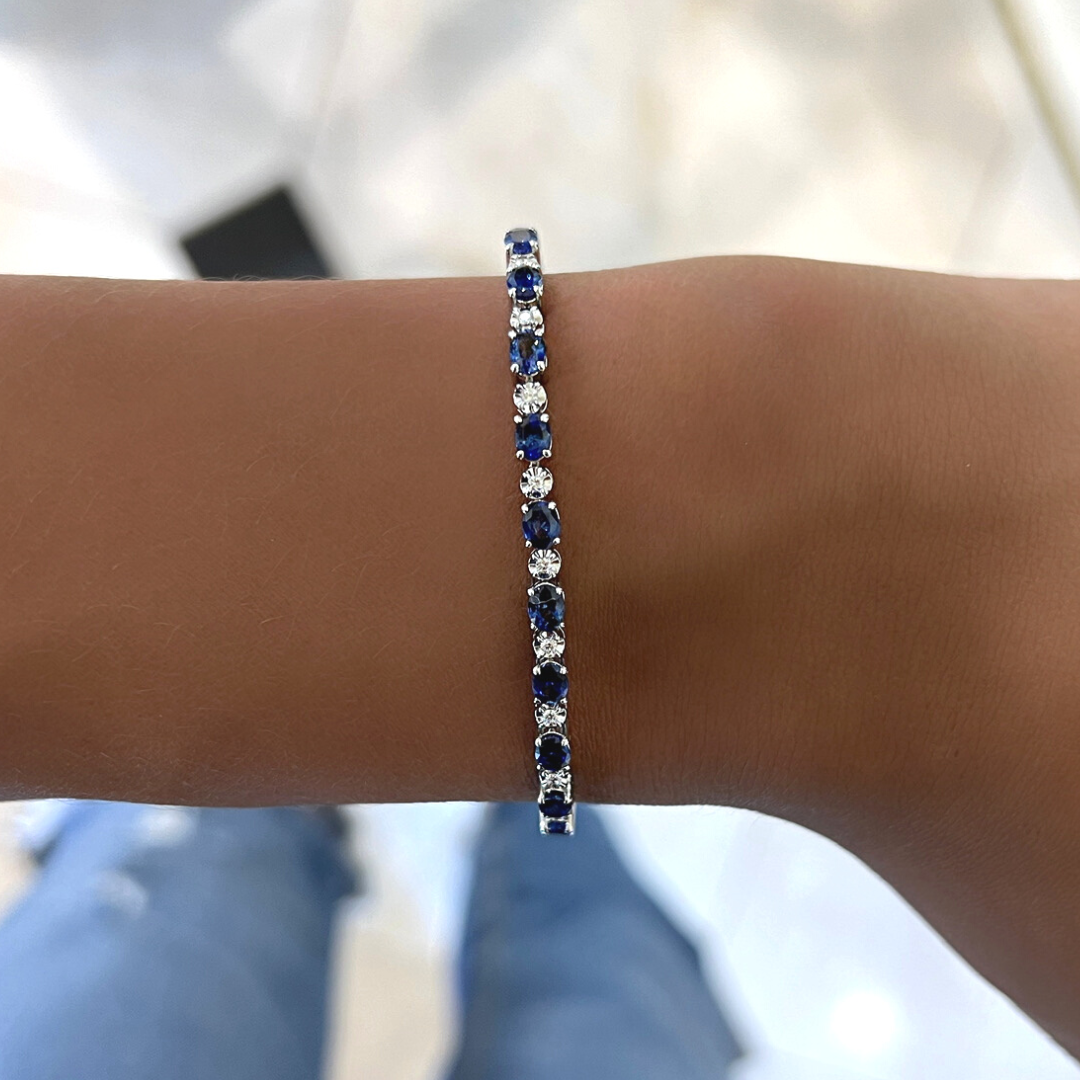This close-up photograph showcases a thin, delicate bracelet encircling a slightly tan wrist adorned with fine, almost white hairs. The bracelet, less than a quarter of an inch thick, features alternating blue and white gemstones, resembling sapphires and diamonds, set in a silver metal—possibly white gold or platinum. The blue stones are oval-shaped while the white ones are perfectly circular, each securely fastened by four prongs. The background, taken during the daytime, is brightly illuminated and slightly blurred, revealing the legs of the bracelet's wearer in medium blue denim jeans with a rip on the left leg. Also visible is the top portion of a phone, hinting at a first-person angle from which the photo was captured.